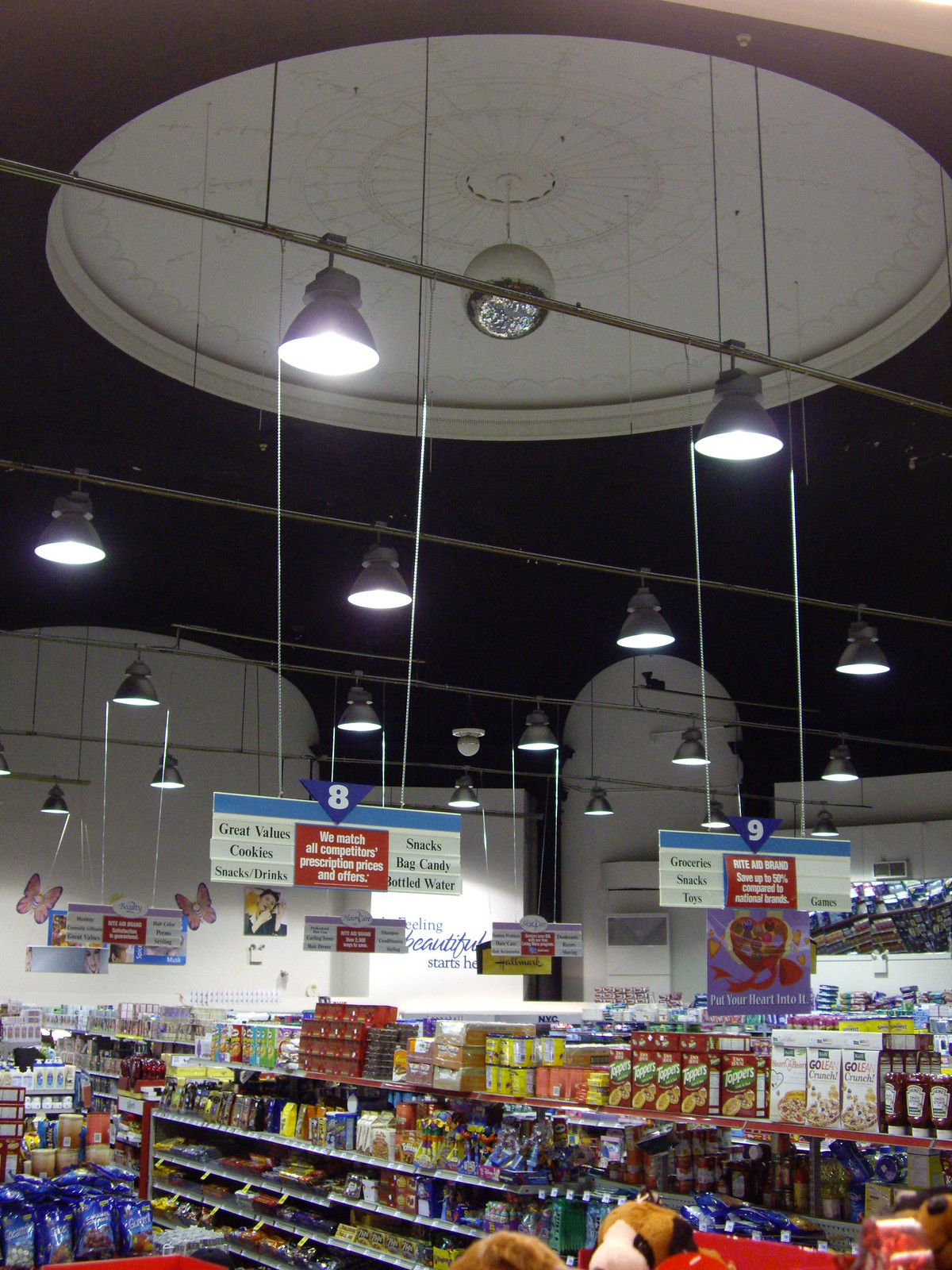This color photograph captures an elevated view within a grocery store, giving the perspective of standing atop one of the aisle shelves. The high ceiling features a distinct circular recess housing a round, white ball-shaped light fixture. Silver horizontal rods, seemingly angled due to the photo's perspective, stretch across the ceiling, suspending white metal-shaded lights that illuminate the aisles below.

Hanging from these rods are various signs indicating aisle contents. Prominent in the center of the image, an inverted blue triangle denotes Aisle 8, featuring a white number eight. This sign, split into two sections, lists items such as "Great Values, Cookies, Snacks, Drinks" on one side, and "Snacks, Bagged Candy, Bottled Water" on the other. A similar sign for Aisle 9, also with an inverted blue triangle and a white number nine, is visible to the right. It lists "Groceries, Snacks, Toys" on one side and "Games" on the other. Both signs feature a red square in the middle that advertises competitive prescription prices.

The shelves below are stocked with various food items like dry goods, canned goods, and snacks. On the bottom right-hand corner, a partially visible shopping cart with red elements contains a couple of stuffed animals. Also seen are two decorative butterflies positioned toward the back. The overall image, enriched in color and details, emphasizes the organized abundance typical of grocery store aisles.